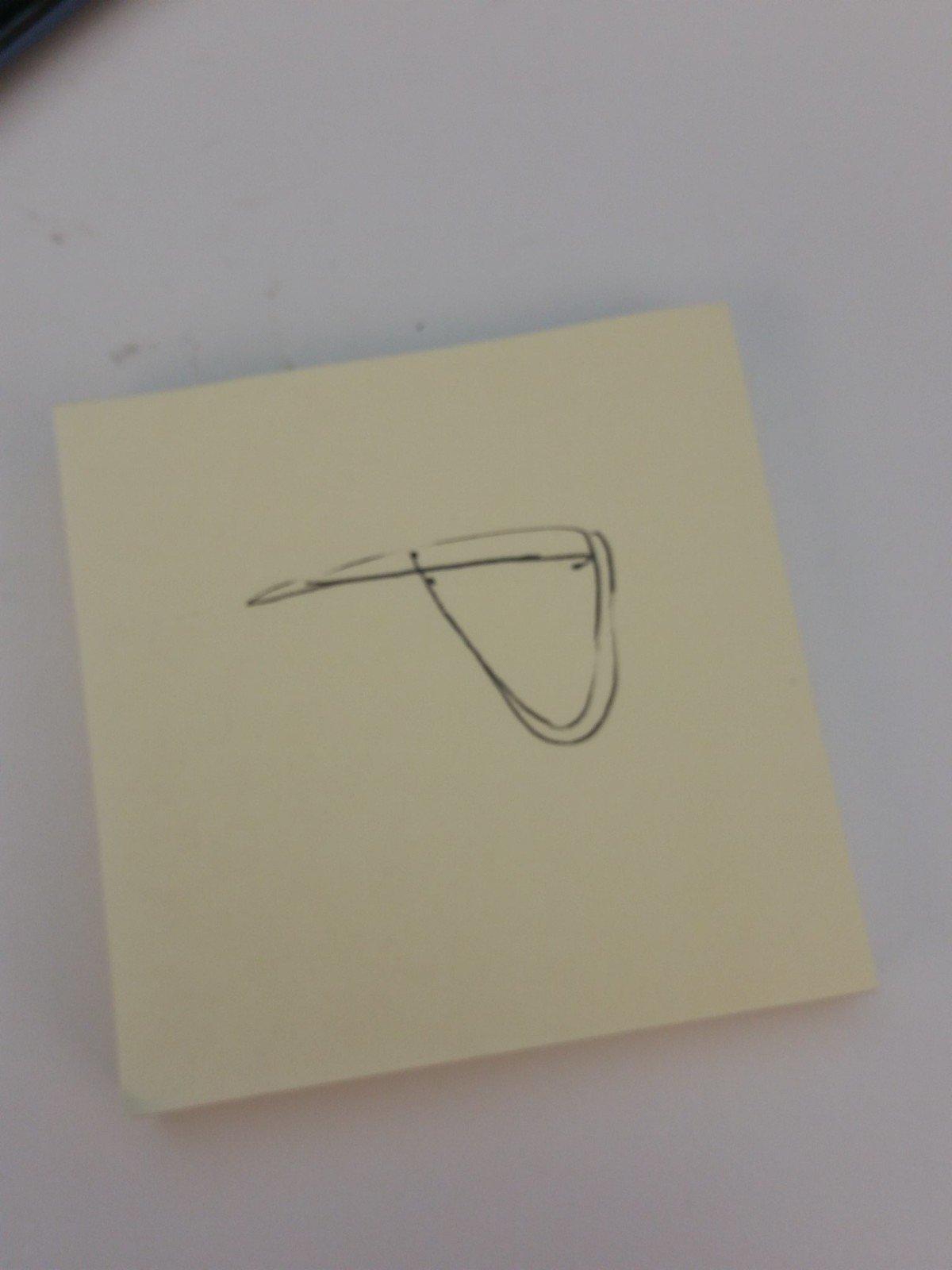A single yellow sticky note dominates the frame, positioned against a neutral background. The sticky note is from a classic 3M pad, identifiable by its familiar hue and slight shadowing around its edges, indicating the pad's thickness. At first glance, it appears the sticky note has been rotated; the quintessential bulge of the letter 'P' faces downward, with the vertical stroke positioned horizontally along the top. 

On closer inspection, the capital 'P' drawn on the note isn't typical; it's creatively stylized. The vertical line of 'P' is rendered as a narrow rectangle filled with parallel lines, culminating in a pointed end. The curved part of the 'P' swoops from the top, gracefully turning a corner before looping back to connect with the rectangle, adding an extra dimension of texture. Shadows create a soft outline around the sticky note, except along the top and right edges, emphasizing the note's three-dimensional aspect. This detailed composition elevates an ordinary sticky note into an intriguing subject of visual interest.